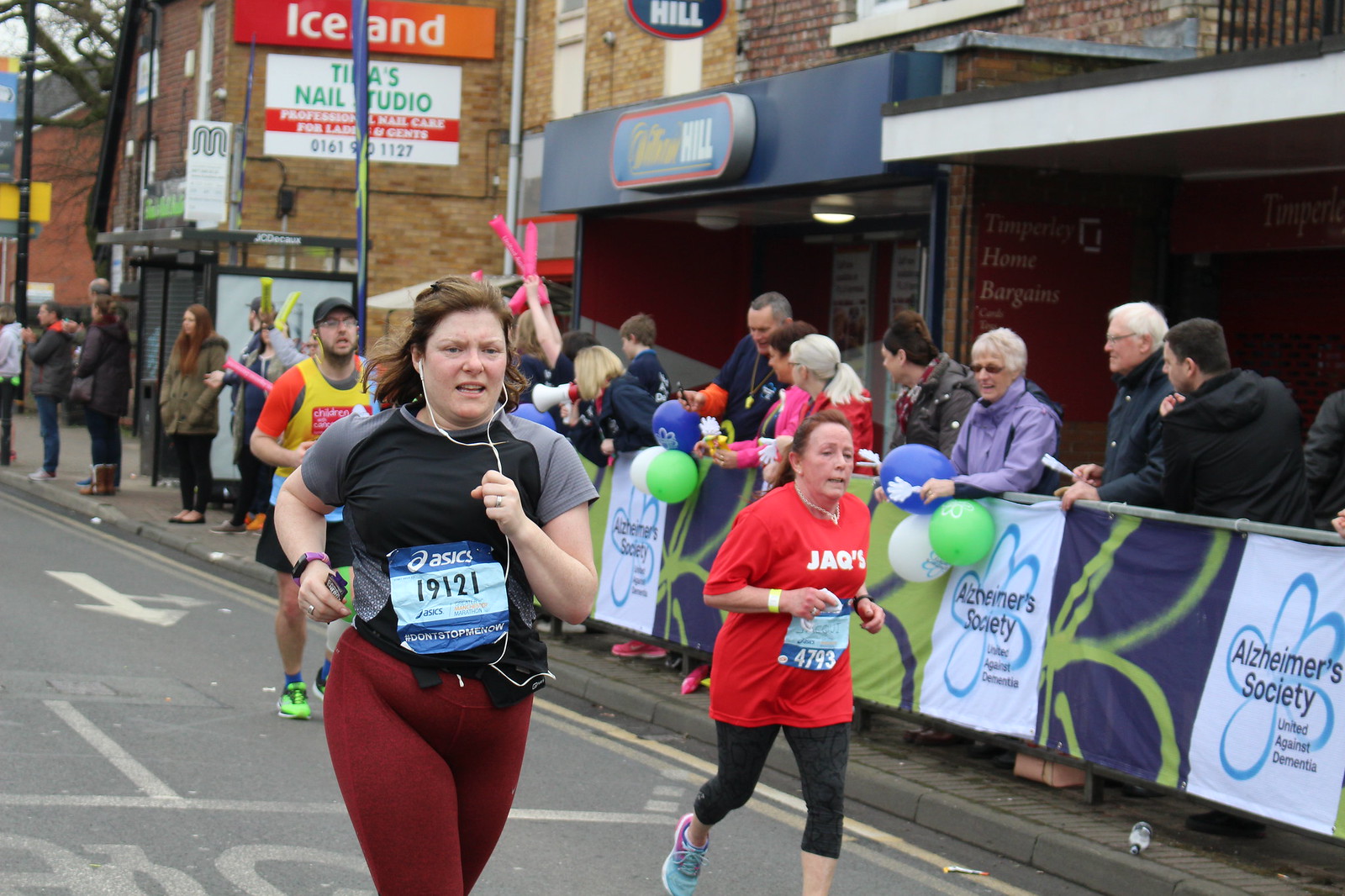In this wide rectangular image of a road race taking place in an urban area, we see a gray paved road marked with white and yellow paint, visible from the top middle to the bottom right corner. Flanking the road is a gray elevated sidewalk lined with a large silver gate, where groups of spectators stand behind banners that read "Alzheimer's Society United Against Dementia." Above these banners are tapestries showing a blue and green painting.

Dominating the scene slightly to the left of center is a white woman with long dark dirty blonde hair flowing back as she runs. She wears white earphones, burgundy-colored leggings, and a black and gray short-sleeved shirt, with the number '19121' on a sign at her waist. To her right, another female runner with long brown hair sports a red t-shirt with "Jack's" inscribed on it, paired with black capri leggings. Also visible is a male runner in the background, identifiable by his baseball cap, neon yellow shoes, black shorts, and a yellow tank top over an orange short-sleeved shirt.

The background reveals an urban setting with old brick buildings displaying various signs, including one with white text on an orange background reading "Iceland" and another below it advertising "Telia's nail salon." Spectators holding balloons lean against the fence, creating a lively atmosphere as they cheer on the runners.